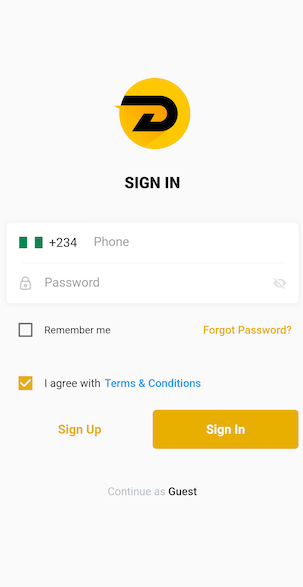The image depicts a user interface for a login or registration page. At the top left, there is a yellow circle with a black letter "D" inside it. Below this are two green squares followed by the number "234" resembling a phone number pad. A padlock icon is displayed next to a password input field which includes an eyeball icon with a line through it to indicate password visibility toggle.

Underneath, there is a checkbox labeled "Remember me" situated next to an "forgot password?" link, highlighted in an orange box with a white checkmark. This section appears in an orange color.

Further below, you see a confirmation message "I agree with terms and conditions," which is blue. There are two buttons: "Sign up" in orange and "Sign in" in white with an orange border around it. Additionally, there is a "Continue as guest" option in gray text.

Overall, the background of the page is a neutral gray, creating a minimalist and clean aesthetic.